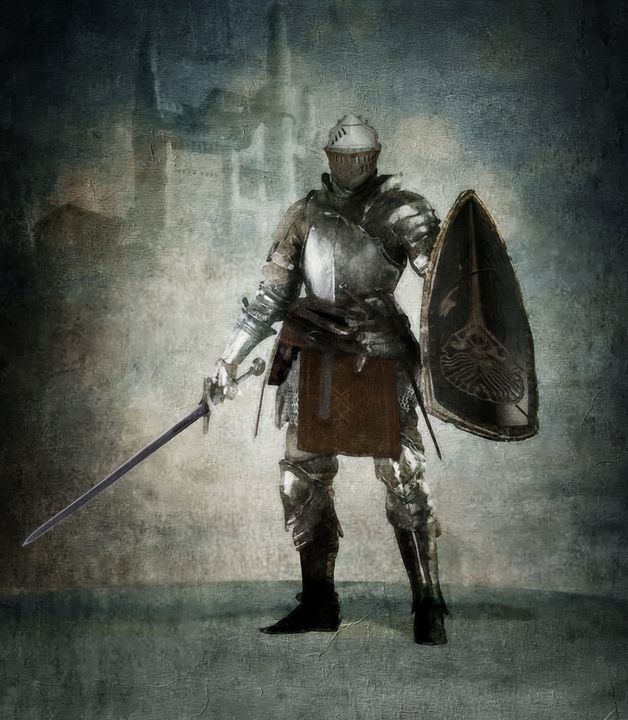This painting depicts a fully-armored knight standing on a vague, gray floor with a shadowy castle featuring a turret in the indistinct background. The main focus is on the knight, who is clad in traditional silver chainmail and armor, covering every part of his body including silver knee guards and tall black boots. His head is protected by a helmet with a face shield, rendering his features unseen. The knight's left hand holds a large black shield bearing an indistinct symbol at the bottom, while his right hand grips a drawn sword. Around his waist, various items, possibly additional weapons in scabbards, are held by a brown utility belt. The painting is dominated by dark, gray, and beige hues that fade into lighter tones near the bottom, enhancing the mysterious aura of the setting.